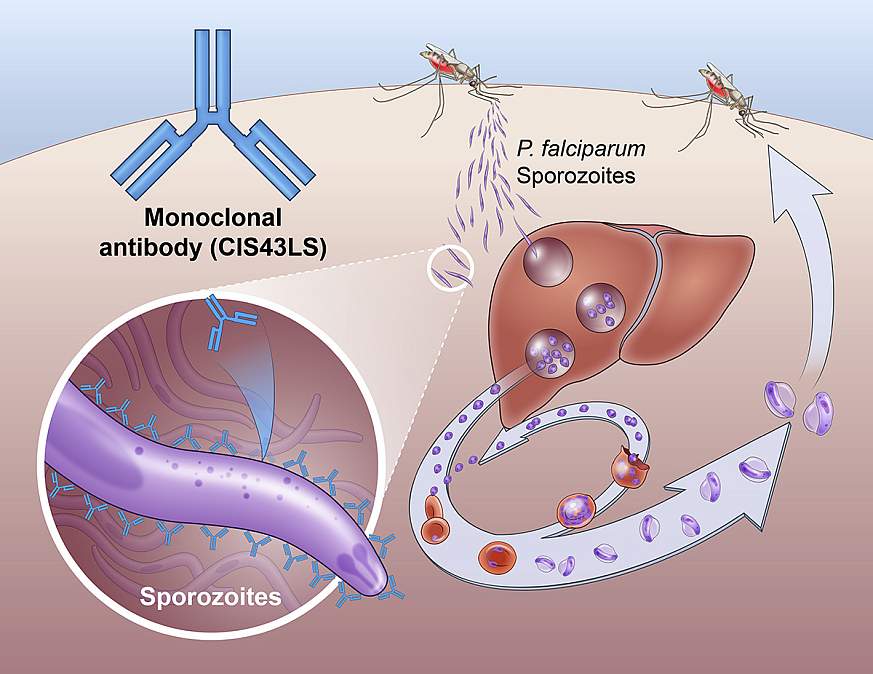The scientific diagram depicts a cross-section of human skin in beige to pink tones. On the skin surface, there are two mosquitoes, depicted with brownish translucent bodies, black legs, beady black eyes, and long thin antennas. Their abdomens are shown in red, indicating they are feeding on blood. One mosquito is injecting something into the skin, represented by thin purple lines with dots inside them, identified as Plasmodium falciparum sporozoites.

A magnified section highlights three sporozoites, enclosed within a white circle, showing their purple, slug-like structure. These sporozoites are surrounded by blue monoclonal antibodies labeled as cis-43-ls, which resemble a triangular or tripod shape with prongs.

To the right of the diagram, an illustration shows the lifecycle of these sporozoites entering and subsequently emerging from the liver. The liver is depicted in dark brown with clear bubbles inside, containing purple cysts or buds, indicating the sporozoites' development. A white arrow illustrates the cyclical process of sporozoites entering the liver, developing, and then re-entering the bloodstream, ultimately to be picked up by another mosquito, perpetuating the cycle.